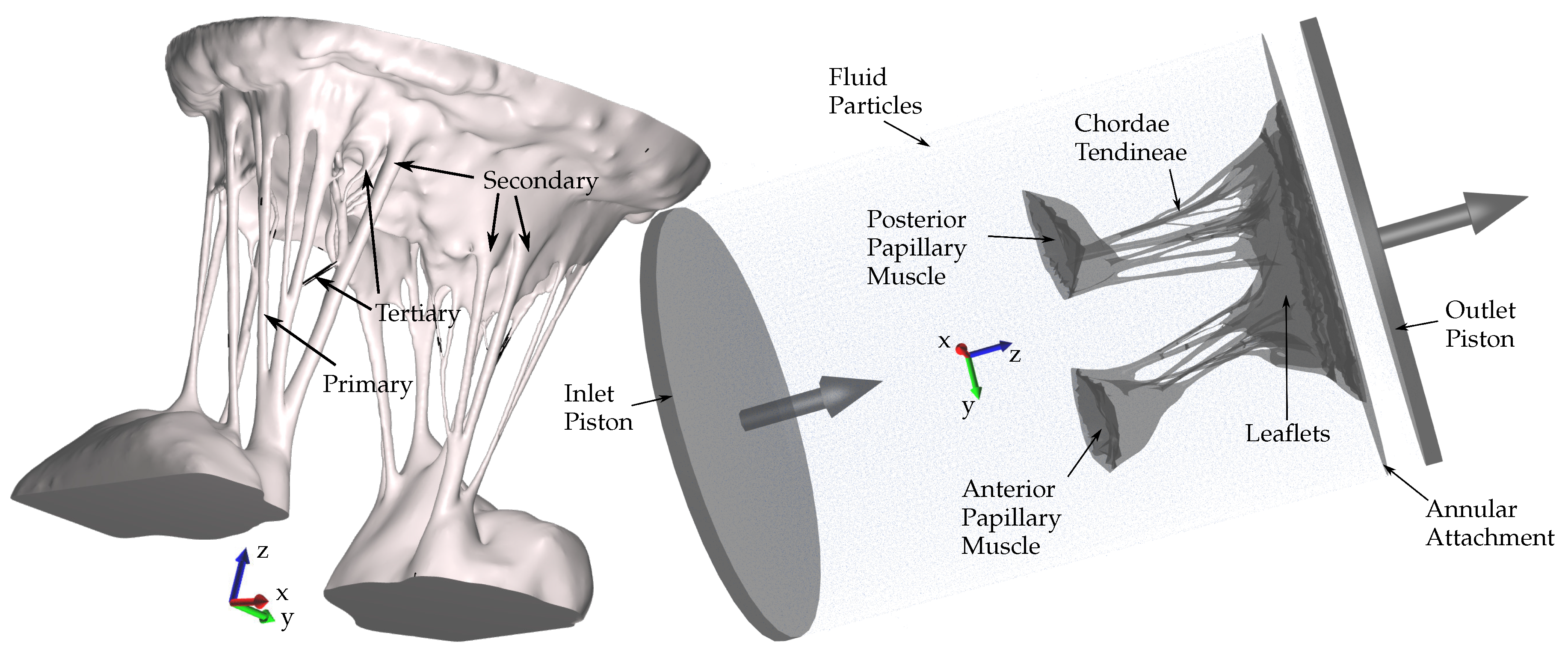This is a detailed, horizontally aligned, gray and black hand-drawn sketch that appears to be from a biology or science textbook, explaining parts of a mammal or possibly human muscles and connective tissues. The image features a primary mass of flesh in grays and pinks on the left side, which extends downwards in a stringy texture resembling melted cheese, dividing into two smaller masses on the top and bottom. The larger top mass and the smaller bottom masses are shaded with gray on their lower parts.

The diagram is annotated with blue, red, and green arrows pointing in various directions (blue up and right, red directly right, and green right and down), labeled with the letters Z, Y, and X. Labels in small black font (Times New Roman) annotate different parts: "Primary" points to the stringy substance on the bottom left, "Tertiary" with arrows to the left and above, and "Secondary" on the top right pointing to the left and below.

The upper section includes a gray disc labeled "Inlet Piston," positioned at an angle with an arrow pointing from its higher left side. Nearby, the same structure is shown turned on its side with annotations for "Chordae," "Tenende," "Fluid Particles," "Posterior Papillary Muscle," and "Anterior Papillary Muscle," with corresponding arrows. There's a noted gray area labeled "Outlet Piston" at the bottom right corner, surrounded by additional labels and arrows.

A horizontally aligned, but slightly diagonal line labeled "Leaflets" runs across, resembling the pelvic area when viewed on its side. Parallel to it, a thicker, black horizontal line labeled "Annular Attachment" runs beneath with a gray arrow pointing out to the right.

The entire drawing is surrounded by labels pointing to different parts, with a slight fuzzy blue background behind the right image. The detailed sketch appears to illustrate the anatomical structure and connection of specific muscles and tendons, despite being somewhat difficult to decipher.